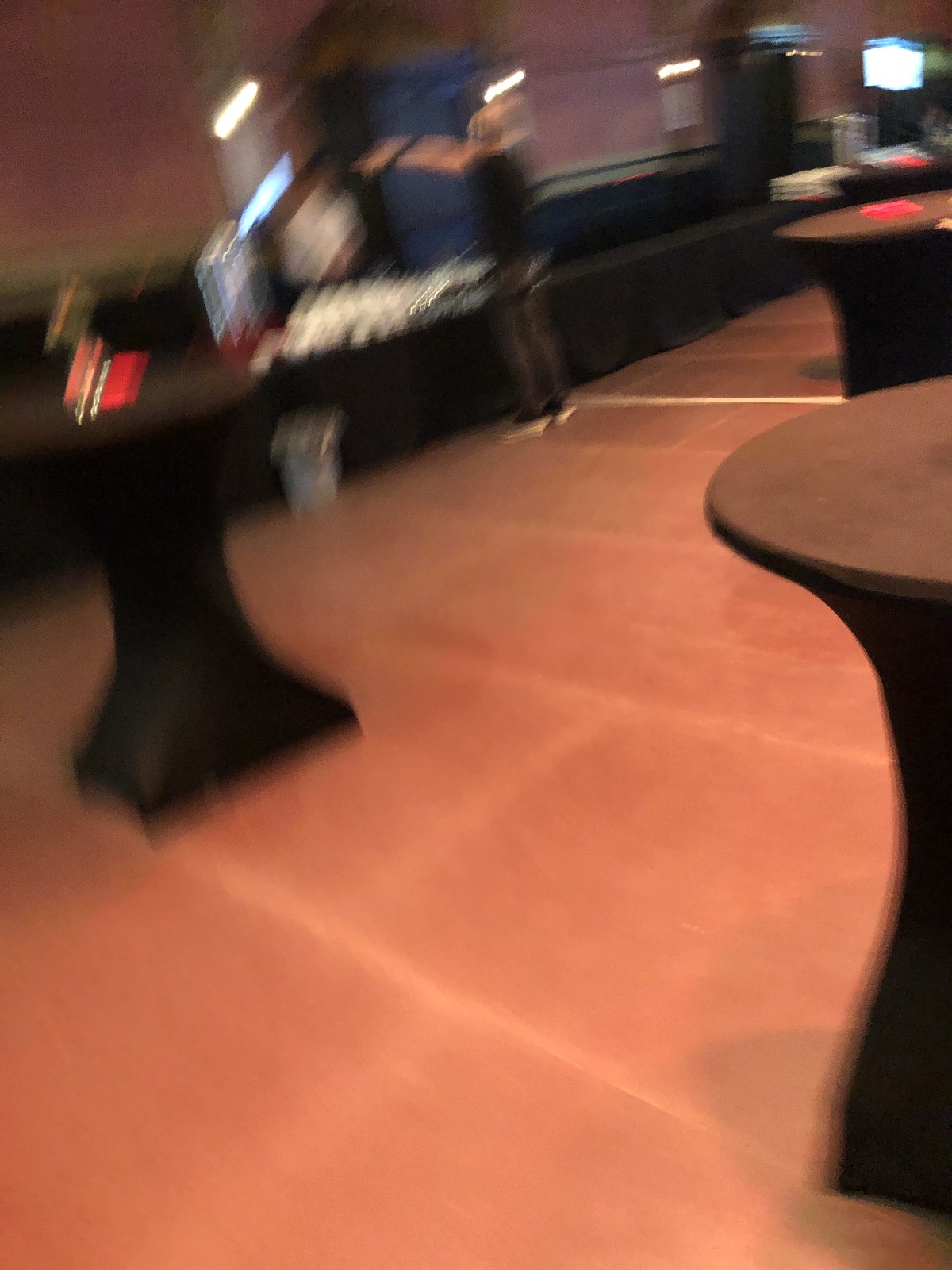The image depicts a room with a brown floor and three round brown tables, each supported by a square base. To the left, there is a red object accompanied by a white and black item. Nearby, a pile of white objects is visible. A person wearing a white shirt is present, standing near a white bucket on the floor. Another individual, dressed in black pants and a white shirt, is pointing at something and has a black device on their wrist. 

The wall in the background is maroon, adorned with three white lights. Below these lights, there is a black shelf-like structure, and to its side, a large square white light mounted on a black fixture. A white object is placed on the counter alongside a white and red item. 

One of the round tables features a red item at its center. There are two white lines on the floor, one across the front and another across the back of the room. A blue cabinet is positioned against the back wall, with a brown object resting on top. Additionally, a white object is located under one of the wall-mounted white lights.